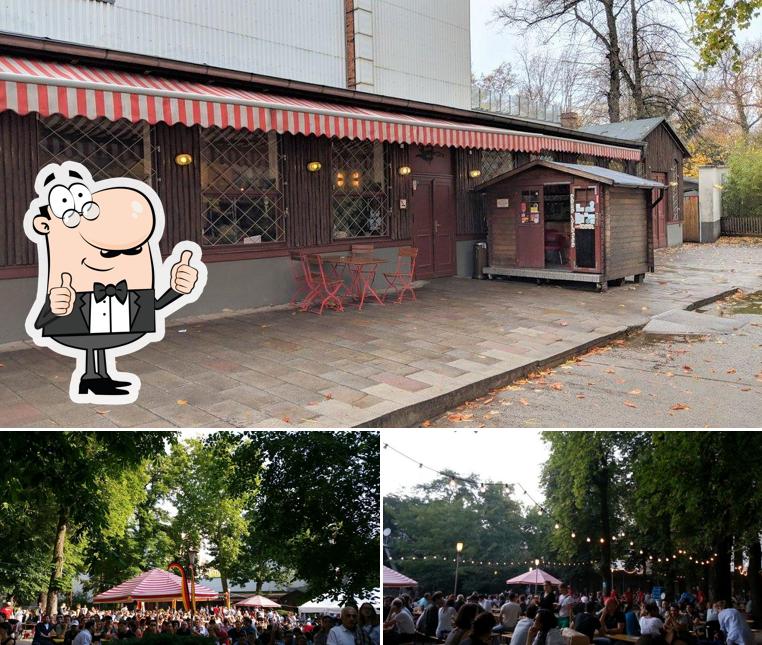The image is a composite of three distinct photos, divided by thin white lines into two top and one larger bottom section. The top left photo shows an outdoor clothing market against a white stone building adorned with black, red, and yellow German flags and awnings. In the foreground, a sidewalk with people walking past a circular clothing rack filled with various garments is visible. The top right photo captures a wooded picnic area with large trees growing through openings in a expansive deck, surrounded by numerous picnic tables and people. The bottom photo depicts a bustling park scene with multiple tent canopies sheltering groups of people. Additionally, on the left side of the bottom section, there's a cartoonish character with an oversized head, small body and legs, wearing a tuxedo and a bowtie, glasses, and sporting a raised eyebrow and mustache, giving two thumbs up.